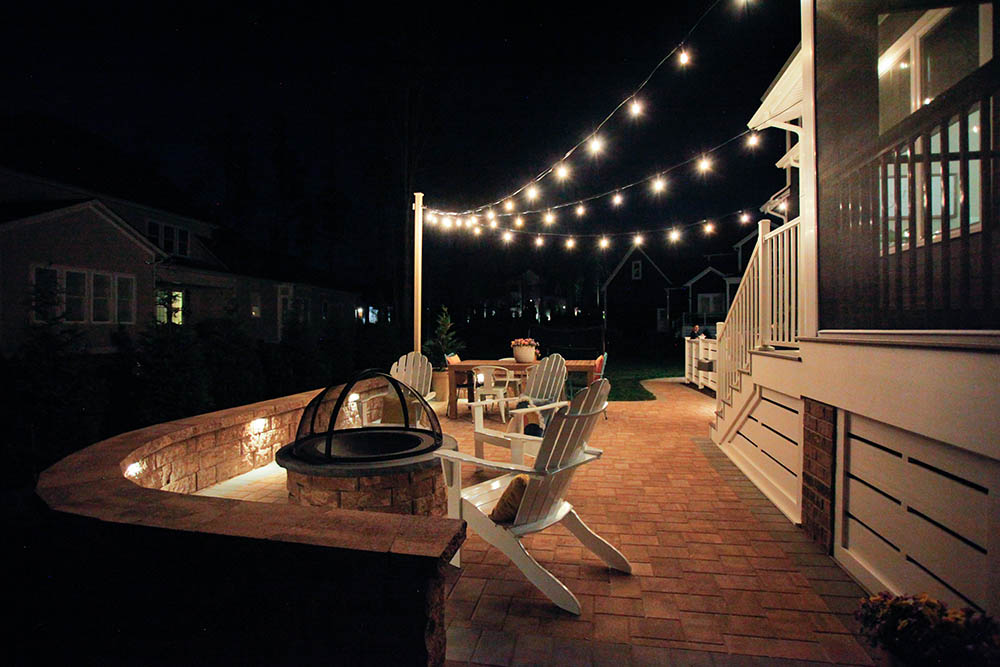This is a photograph taken at nighttime, showcasing a meticulously designed backyard space, possibly a porch or patio. The primary structure in the image is a white house featuring white wood shingles and glass sliding doors. Access to the main area is provided by a staircase that leads down to a charming brick-paved patio, characterized by its reddish-brick tile flooring. The patio is adorned with inviting white Adirondack chairs, and a table, as well as a fire pit encased in a metal frame.

Hanging above, from a white post attached to the roof of the house, are strands of warm yellow string lights, reminiscent of Christmas lights, adding a cozy ambiance to the setting. In the background, another house is visible—this one is red with white trim, evoking a farmhouse style. The surrounding area appears to be a quiet, residential neighborhood, with only a few lights illuminating the night sky. The overall scene gives a sense of a serene and well-cared-for outdoor living space.